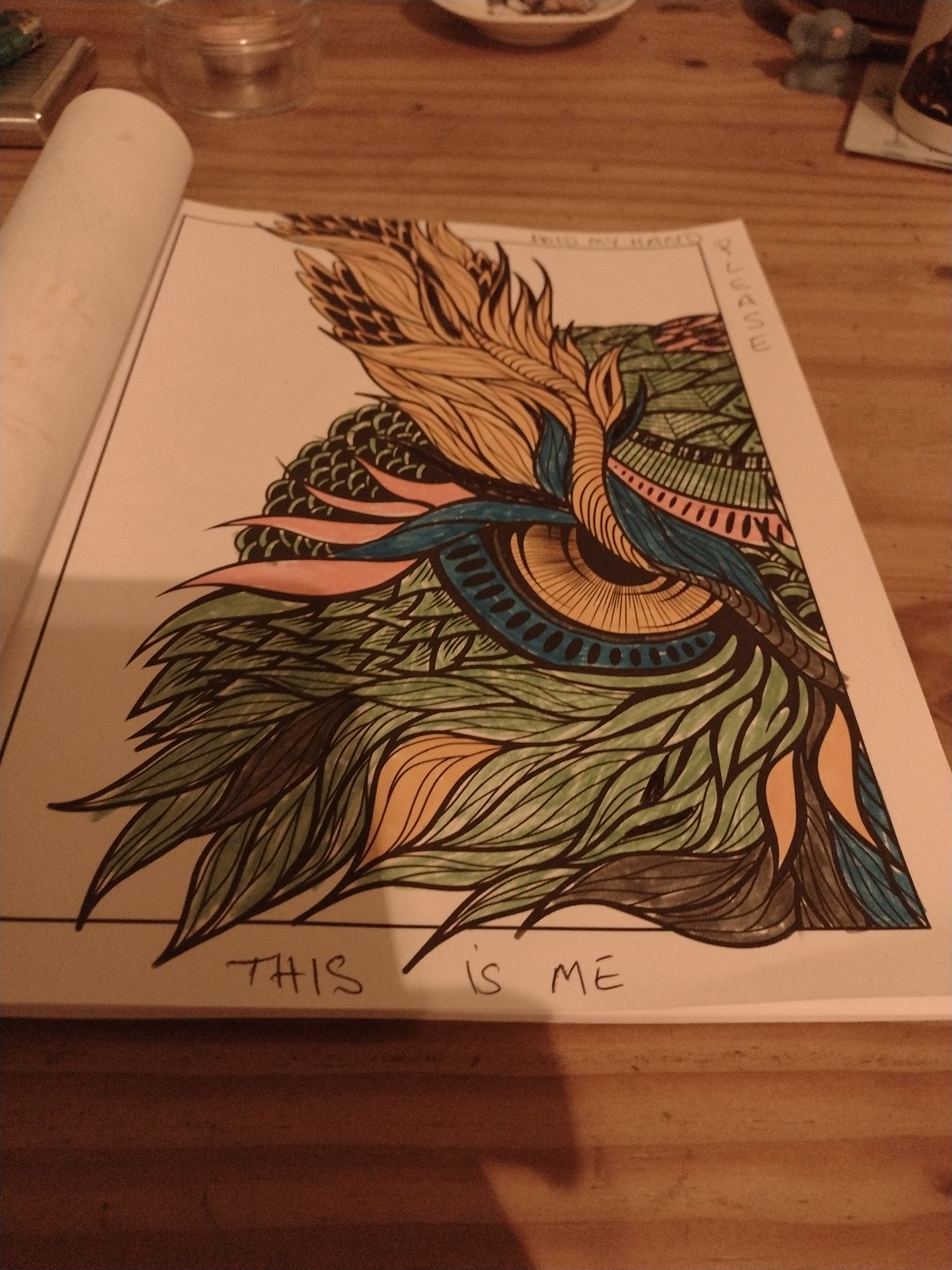An open coloring book rests on the right side of a light-colored wood desk, with its front cover and preceding pages bent back. The focal page depicts the detailed face of a great horned owl, characterized by prominent feather tufts extending from the corners of its eyes. The drawing is colored with a blend of dark blue, forest green, brown, and yellow, complemented by subtle highlights of rust red-pink, forming a palette of muted earth tones. Handwritten words in pen adorn the page—"Hold my hand" at the top, "Please" running down the top right edge, and "This is me" along the bottom edge. 

In the background, a cluttered assortment of objects adds context to the setting: a cigarette case and lighter, a mason jar holding a votive candle, a dirty ashtray, a small elephant figurine, and an indeterminate white object, possibly a coffee mug on a coaster.